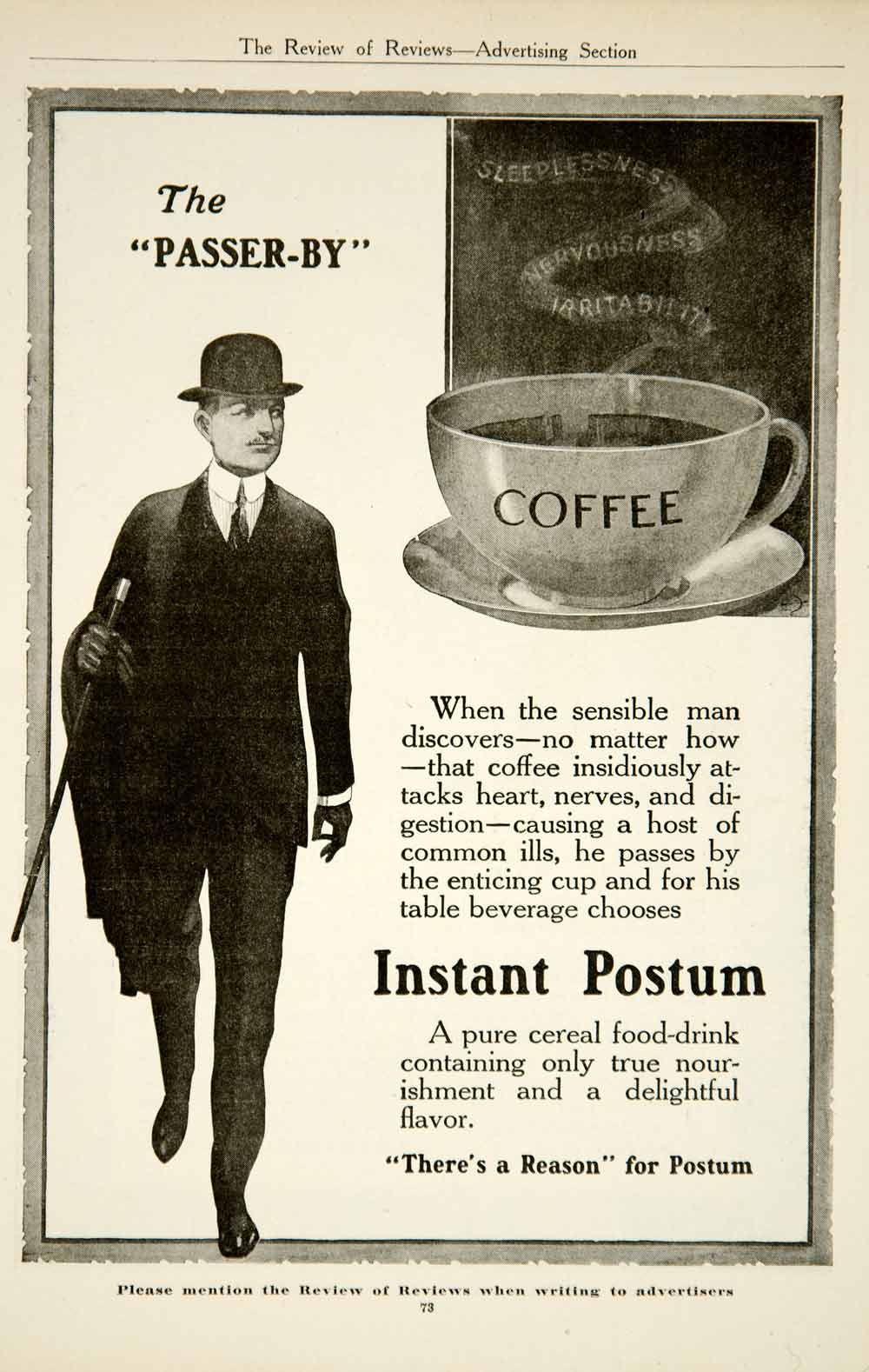This grayscale vintage advertisement, likely from the 1920s or 1930s, appears to be a page from a magazine titled "The Review of Reviews — Advertising Section." Dominated by a dark gray border, it prominently features a well-dressed gentleman labeled "The Passerby." This man, characterized by his dark suit and tie, white shirt, black leather gloves, and polished leather shoes, is complemented by his derby hat, mustache, and a coat draped over his right arm. He holds a walking stick with a white tip, evoking the style of affluent men from that era. The passerby is depicted in motion, looking to the side, and seemingly ignoring a large cup of coffee illustrated to his right. The cup has the word "coffee" inscribed on it, with steam forming the words "sleeplessness," "nervousness," and "irritability" to emphasize the negative effects of coffee. Beneath the image, the text reads: "When the sensible man discovers, no matter how, that coffee insidiously attacks heart, nerves, and digestion, causing a host of common ills, he passes by the enticing cup and for his table beverage chooses Instant Postum, a pure cereal food drink containing only true nourishment and a delightful flavor. There's a reason for Postum." The ad concludes with a note: "Please mention The Review of Reviews when writing to advertisers." A page number, "73," is displayed at the bottom.